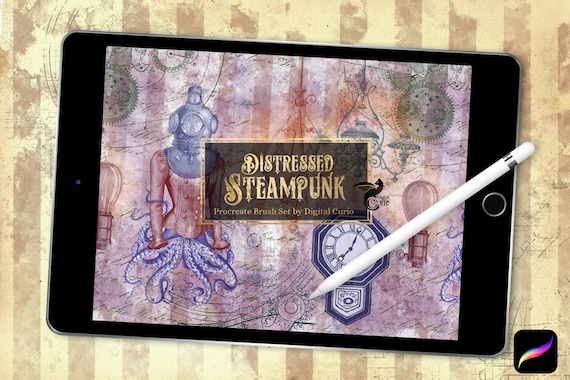The image features a drawing tablet positioned in the center against a beige and tan striped background with perpendicular stripes. The tablet is encased in a black frame and oriented in landscape mode. Across the screen of the tablet lies a white stylus with a silver band near the top, positioned diagonally from the top right to the bottom left.

Displayed prominently on the tablet screen is a label that reads "Distressed Steampunk Procreate Brush Set by Digital Curio," alongside a cat with wings symbol, all within a small rainbow-colored box located in the lower left-hand corner. Surrounding this label, the tablet's screen showcases a variety of pastel images including a brown label with yellow and tan lettering, pastel shades of green, pink, a little bit of purple, dark purple, and blue.

Central to the illustration is a woman wearing a dress with octopus tentacles for the skirt and a gray steampunk helmet, iconic to the steampunk art style. Additionally, there is an old-style Roman numeral clock indicating the time as 5 minutes past 7, along with muted background elements that resemble gears, hot-air balloons, lightbulbs, and cylindrical shapes, all contributing to the thematic steampunk aesthetic.